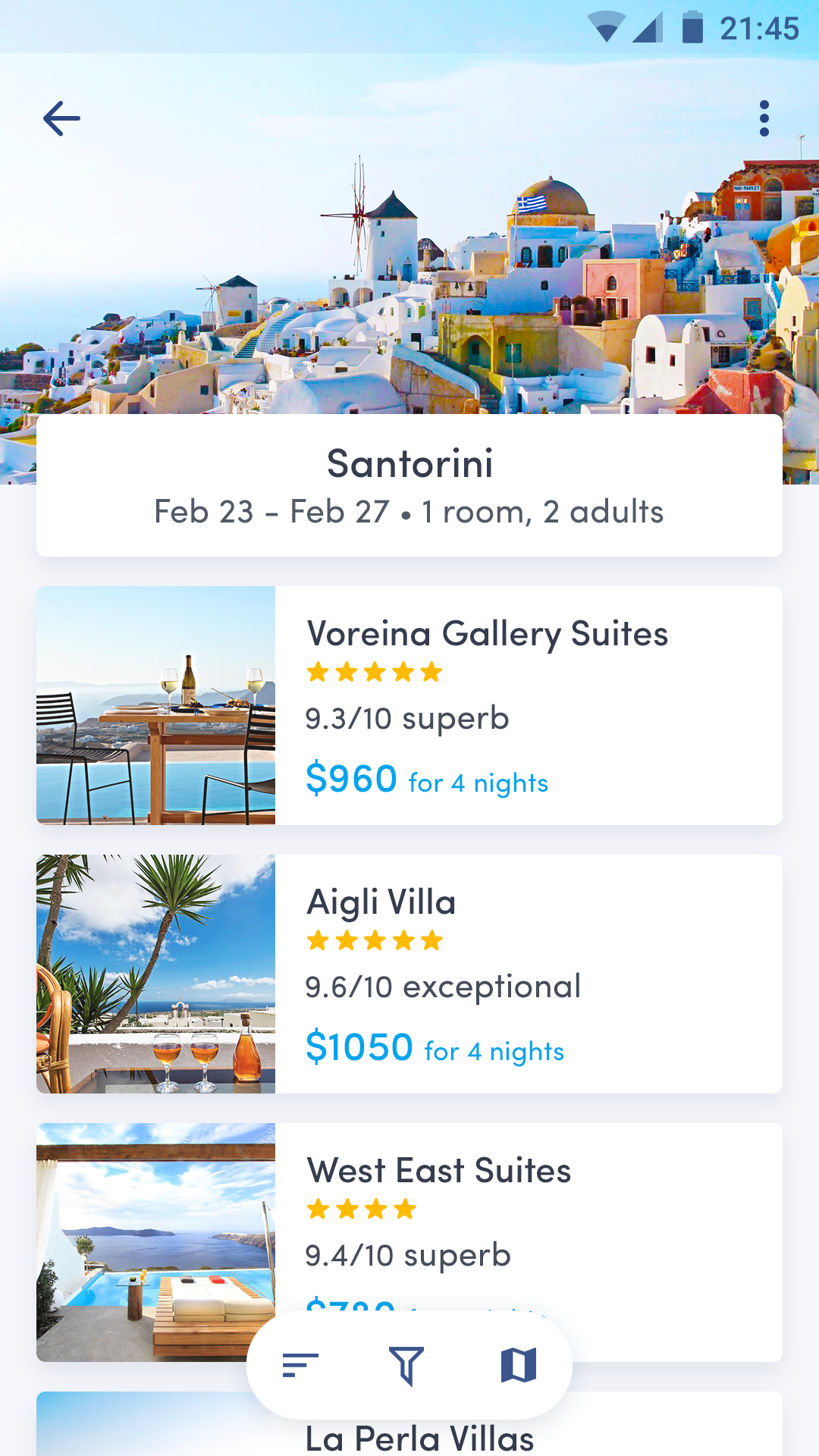This detailed caption describes a screenshot taken on someone’s cell phone. The image showcases a stunning cityscape, possibly of Santorini, with a bright, clear blue sky and water visible in the distance. The city is perched on a hill, with picturesque white buildings dotting the landscape, creating a visually striking scene. 

At the top of the phone screen, the time reads 21:45, and the battery is approximately 90% charged. There are two additional icons next to the battery indicator. An arrow pointing to the left is also visible at the top of the screen, along with three vertical dots, suggesting additional menu options.

Below this, there's text that reads "Santorini February 23rd to February 27th · 1 room · 2 adults," indicating a travel booking. The lower portion of the screen is divided into four sections that can be scrolled through. Each section features a picture accompanied by details such as the star rating, pricing, and other relevant information about the accommodations. The bottommost section is partially cut off due to the size constraints of the screen.